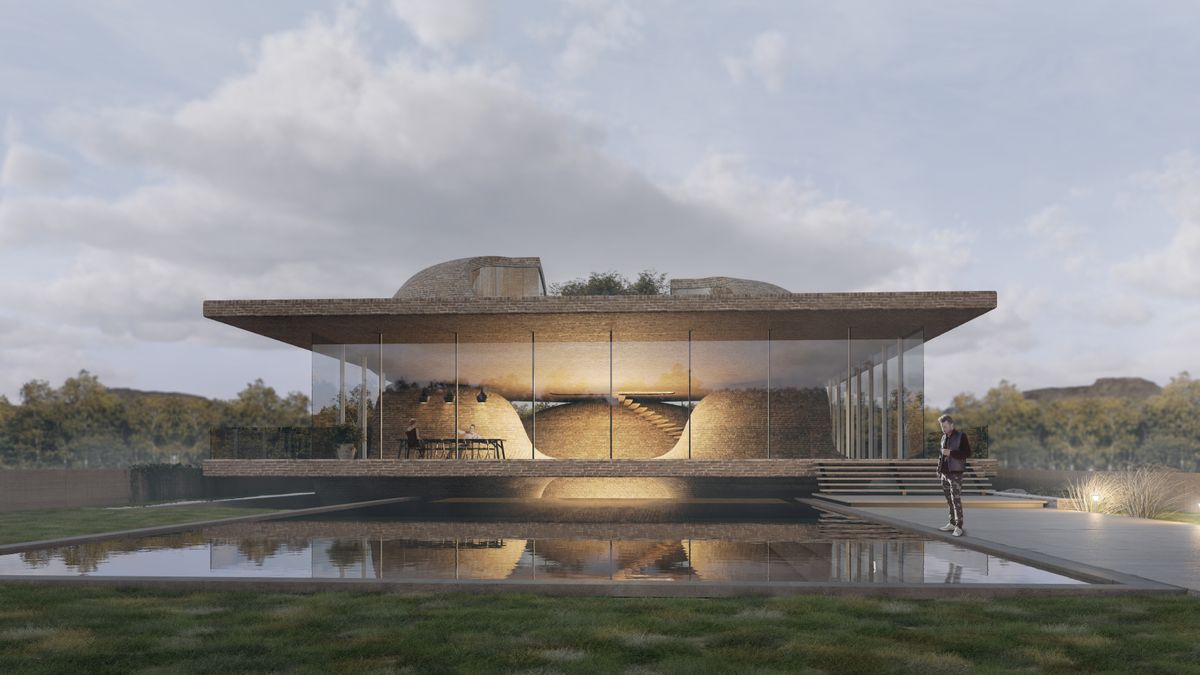This image features a detailed artist's rendition of a cutting-edge, modern building that prominently highlights its sleek design and innovative architecture. The structure is distinctively square and somewhat resembles a sandwich, with two rectangular forms encompassing a central section adorned with extensive windows from floor to ceiling. The tops of these structures crown the building with two half-domes featuring windows.

The house is composed of glass walls on the front, sides, and back, providing a transparent view into the interior. Inside, several stone or brickwork dome-shaped rooms can be discerned, complete with staircases that lead to roof access. The roof itself hosts further dome structures, consistent with the building's unique aesthetic.

In front of the house, a well-maintained grassy area encircles a large, square man-made pool. Adjacent to this pool, towards the right, a person stands on a concrete walkway holding a drink and gazing at the water. This person is situated beside floating stairs that lead to the house, seamlessly integrating with the modern ambiance.

Additional details include a table and chairs inside the house, which is illuminated by studio lights, adding to the sophisticated, gallery-like atmosphere. 

The sky above the house is filled with dramatic gray clouds, enhancing the overall artistic presentation of the image. The entire scene measures approximately six inches wide by three inches high, reminiscent of a colored pencil artwork, effectively capturing the futuristic essence of this architectural marvel.